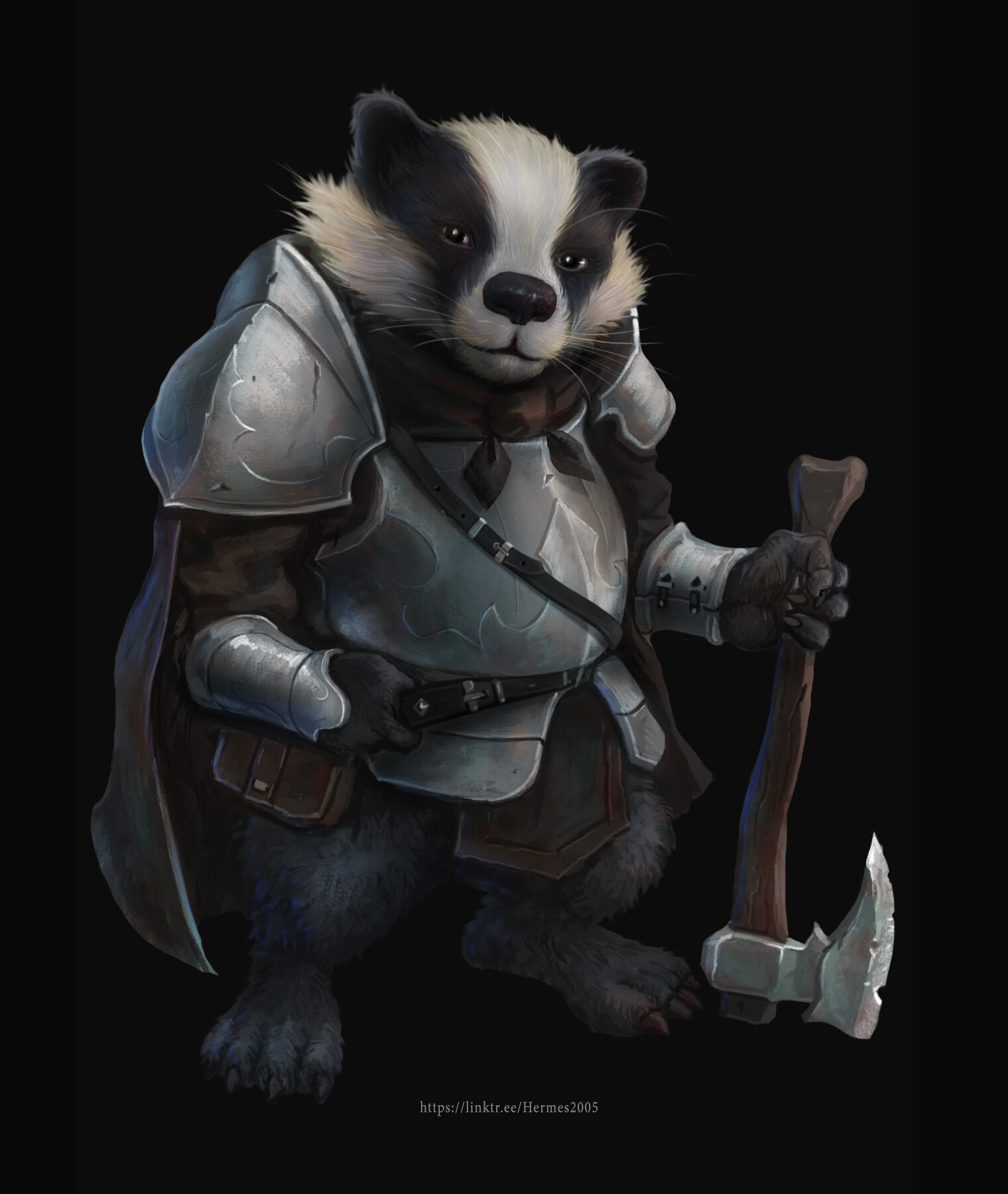This is an image with a black background, featuring a detailed cartoon creature that appears to be a blend of a panda bear with elements of other animals. The creature has distinctive black fur around its eyes, white fur on its face extending from its mouth up to its forehead and beneath its ears. The animal is adorned in knight's armor that covers its chest, shoulders, and forearms, with a brown, bow-tied scarf secured at the front. Additionally, it has a black belt with a knapsack slung across its shoulder, the strap running down to its right waist.

The creature's attire includes both metallic and leather components. The armor is complemented by a brown shirt or cape visible underneath, adding texture to its otherwise armored appearance. Its feet are clawed and left uncovered, revealing a dark gray hue. In its left hand, the creature firmly grips a sharp, metallic axe that is pointed downwards towards the bottom right of the image. The image showcases this intricate, armor-clad cartoon animal striking a formidable pose against a stark black background.